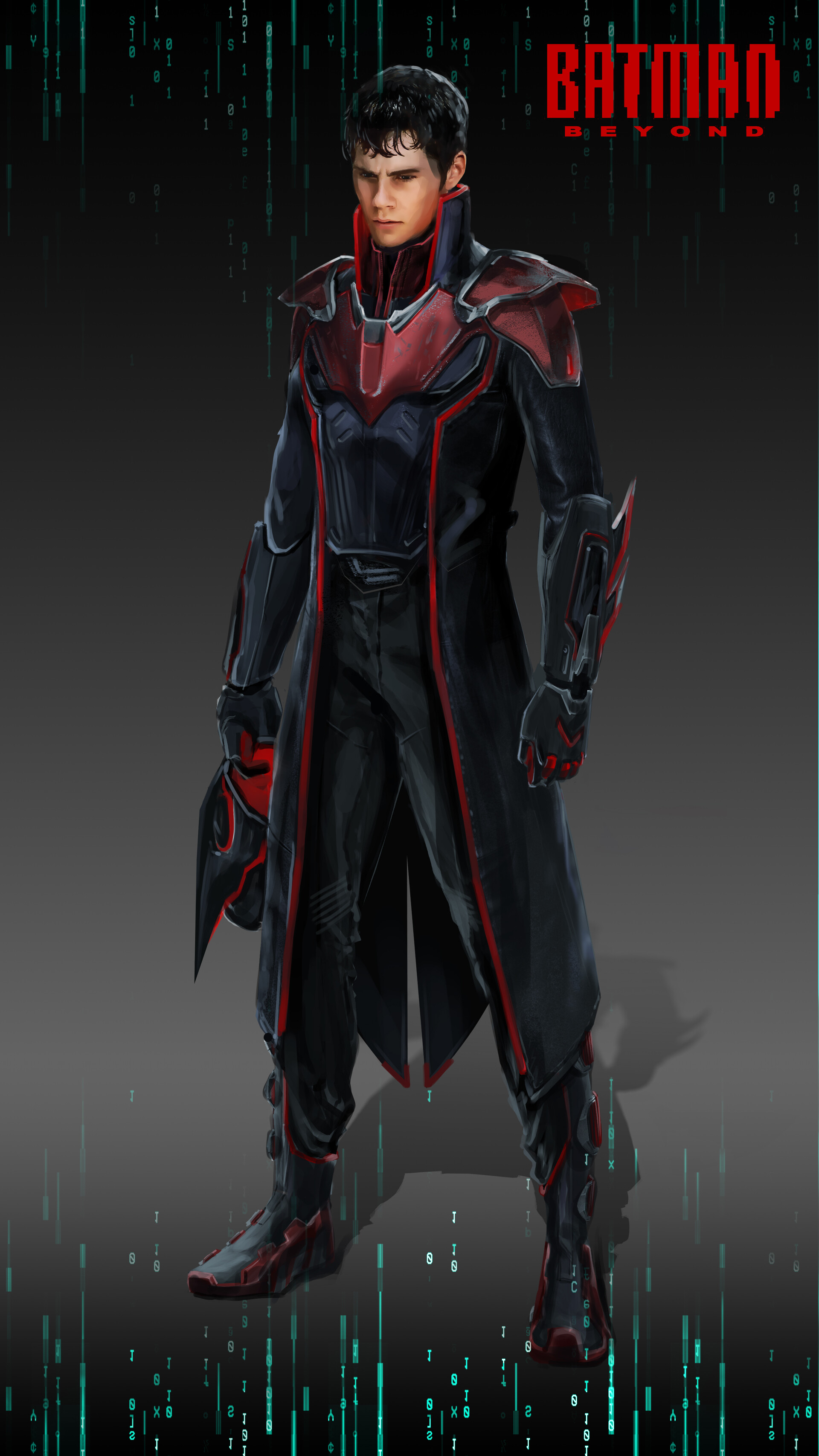This comic-style artwork features a young adolescent man with black curly hair and a dark complexion. He is dressed as a Batman Beyond character, with the text "Batman Beyond" appearing in the upper right corner. The character is depicted looking downward with a focused, serious expression. He wears a black one-piece bodysuit that includes a red and black vest, red-shouldered chest and shoulder plates, and black gloves extending over the elbows. His high-collared, long black coat features red trim and tails with red tips. In his right hand, he holds a black mask with red trim, suggesting his hidden superhero identity. His black boots are embellished with red highlights and small spikes. The background is a combination of black and grey tones, with pixelated green streaks and code-like striations at the bottom and top of the image.